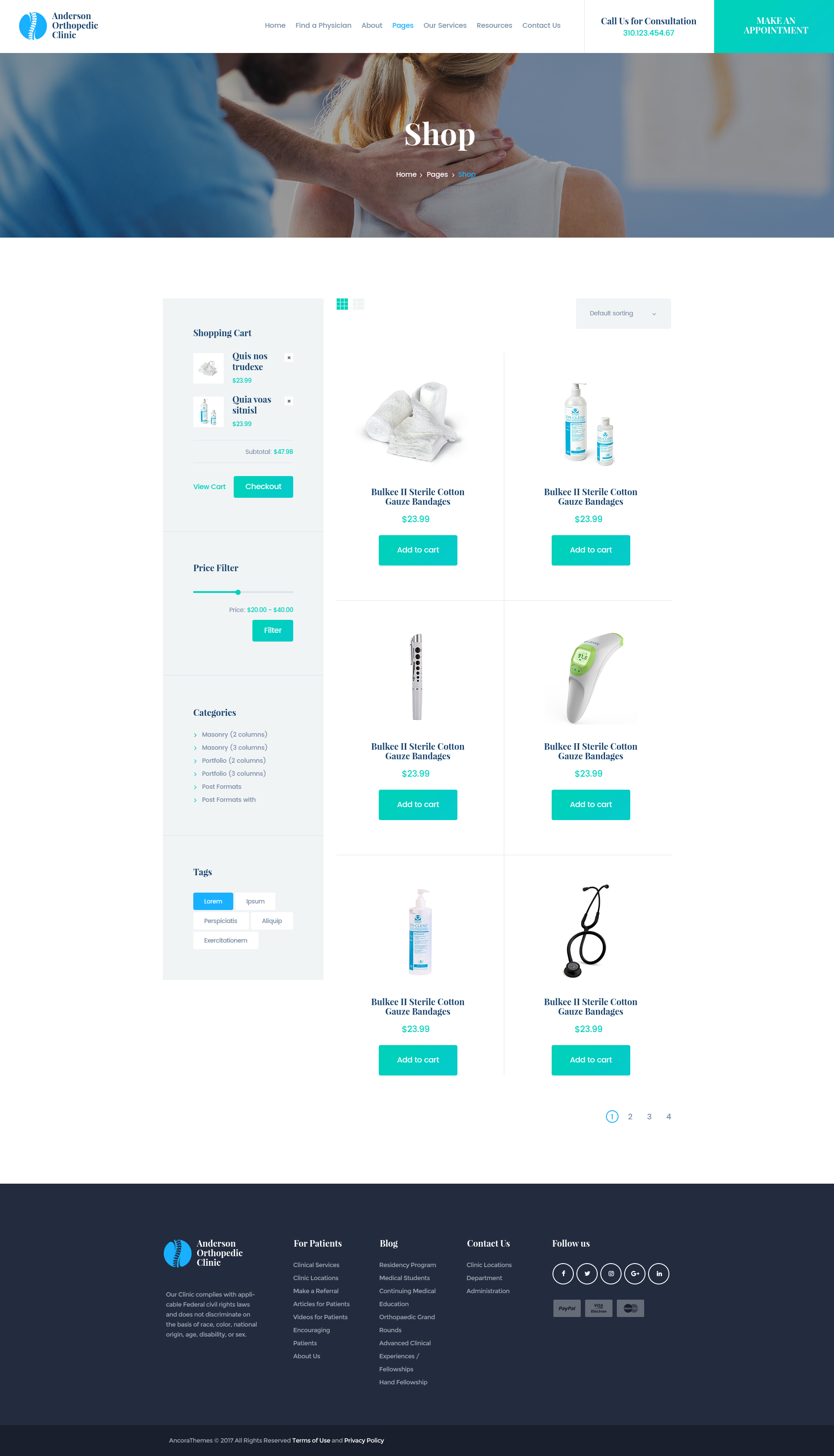This screenshot features a website, albeit in a blurry and small format, making it challenging to read. At the very top of the page, there is a white navigation bar. On the left side of the bar, a blue icon resembling a human vertebra is clearly visible, accompanied by the text "Anderson Orthopedic Clinic" in black font. Towards the right end of this bar, there are clickable selections for different webpages, though the text is too small to decipher. Adjacent to these selections, there is a mention of "Call for cancellation" beside a light blue square containing white text.

Below the navigation bar, there is a prominent photo displaying a Caucasian man, clad in blue scrubs. He has a brown beard and noticeably dirty fingernails. His hand is gently resting on the neck of a Caucasian woman who is wearing a white tank top and has blonde hair styled in a side ponytail. This interaction seems to be taking place in a medical office setting.

Further down the page, there is a section featuring a small shopping cart icon. The items listed beneath this icon appear to be related to medical supplies, which users can presumably add to their cart for purchase.